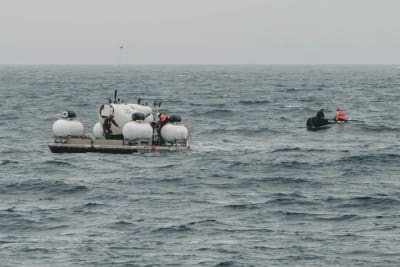This photograph captures a haunting scene of two sea vessels on a choppy, gray ocean. Predominantly muted in hues—gray, blue-gray, and white—accentuated by small black and red details, the ocean dominates the bottom three-quarters of the image. The horizon sits just above this, blending into a solid, overcast sky devoid of clouds or sunlight, suggesting midday under a thick layer of smog or fog. 

To the left side of the image, there is a large, flotation platform that appears to serve as a submersible launch pad. This structure is marked by five large, white, orb-like objects, likely flotation devices or water tanks, and there are several human figures visible on it. Moving to the right of the image, a smaller vessel—a two-person dinghy—features prominently, with one person dressed in black and the other in red. These individuals seem to be making their way toward the larger platform.

The dismal sea and foreboding sense of journey forward give this photograph a somber, newsworthy quality reminiscent of last glimpses of ill-fated marine expeditions.